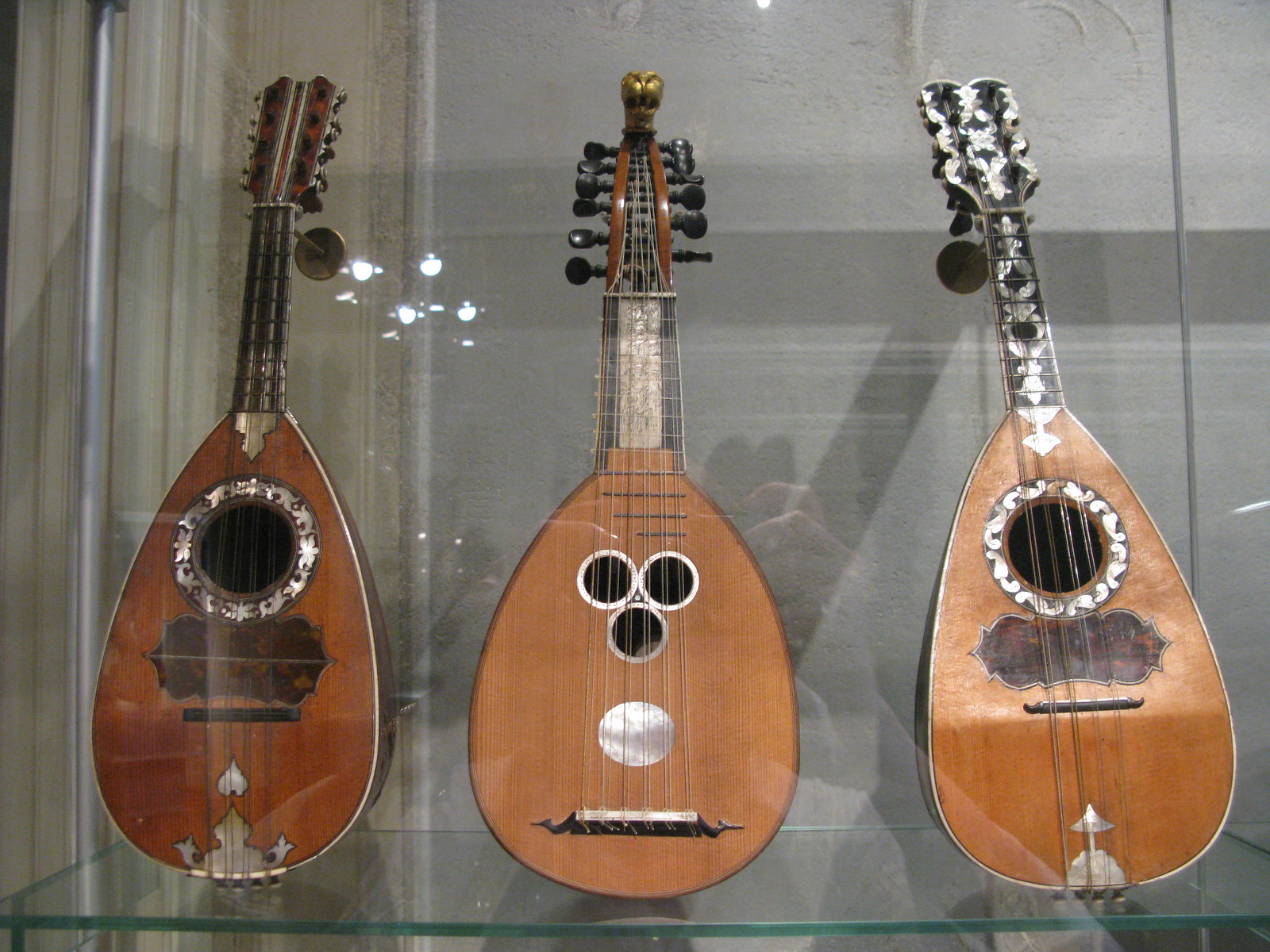In this image, there is a glass display case with a gray background, showcasing three unique stringed instruments that resemble ukuleles but aren't exactly guitars. Each instrument has distinctive features and decorative designs. 

On the left, there is a dark brown instrument with silver decorative elements around its single hole and towards the bottom. Its strings run up to a red fender at the top. 

The middle instrument is a lighter brown ukulele with three holes in the center of the body, a silver circle below these holes, and an array of black knobs on either side of the strings, twelve in total. The strings run up to a golden crown-like top.

The instrument on the right is similar to the one on the left in having a single hole with silver decorations around it, but it also features a silver element running up its struts. This ukulele is lighter in color compared to the one on the left but darker than the one in the middle.

The shapes of the instruments are teardrop-like, with rounded bottoms and short necks. In the reflection on the glass display, the arms and hands of the photographer can be seen, capturing this detailed and carefully arranged exhibit.